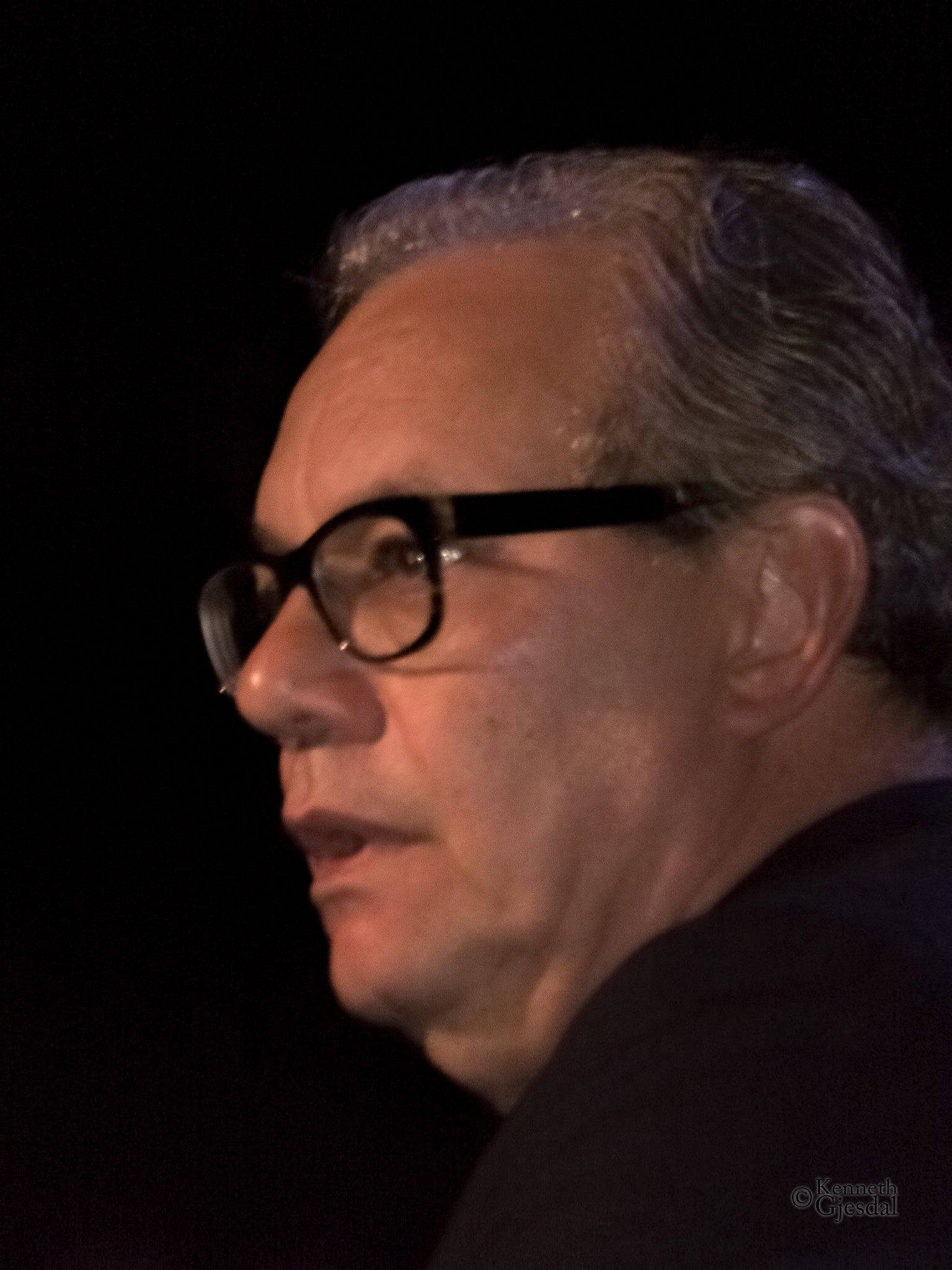This close-up photo captures a middle-aged white man, identified as Lewis Black, an American stand-up comedian and actor. He wears thick black plastic glasses perched near his nose, revealing his likely brown eyes, and short, slicked-back, graying hair. Dressed in a dark shirt that blends seamlessly with the completely black background, Lewis Black appears slightly out of focus as he looks towards the left with a somewhat open mouth, as if about to speak. His expression conveys a sense of concern. The image features text in the bottom right corner reading, "copyright Kenneth Gjestdal," with "G" capitalized and the rest in lowercase against a white shadow. The overall color palette of the photo is predominantly black, gray, and tan.